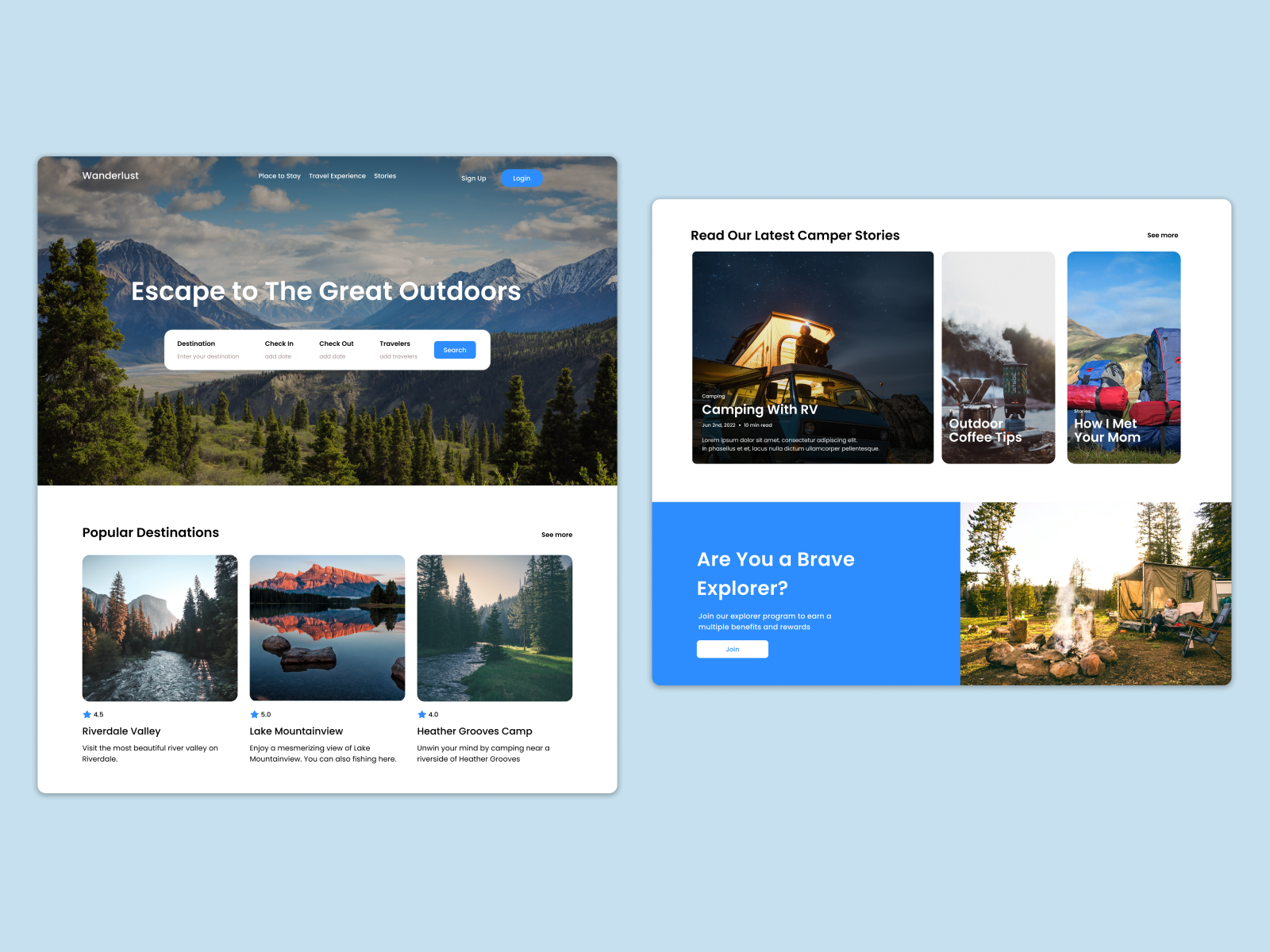In this image, the screen is divided into smaller sections against a light bluish background. On the left side, the top left corner features the word "Wanderlust" in bold white text. In the top middle section, three categories are listed, also in white text, though they are hard to read. The top right corner includes the options "Sign Up" and "Log In" with white text; "Log In" is highlighted with an oval-shaped blue background.

Centered in the middle of the left section, the phrase "Escape to the Great Outdoors" is prominently displayed. Below this, there is a rectangular shape containing some information that is too small to read. Further down, the text "Popular Destinations" appears in black, followed by three square boxes. 

The first square, labeled "Riverdale Valley," features an image of a river flanked by trees under a clear sky. The second square, labeled "Lake Mountain View," displays a reflective, clear lake with mountains mirrored in the water. The third square, labeled "Heather Groves Camp," showcases a grassland with large, vibrant green trees.

On the right side of the image, the text "Read Our Latest Camper Stories" is visible. Below this, three article titles are listed: "Camping with RV," "Outdoor Copy Tips," and "How I Met Your Mom."

This detailed layout suggests a website or digital platform dedicated to outdoor adventures and camping experiences, offering both inspiring destinations and useful tips for outdoor enthusiasts.